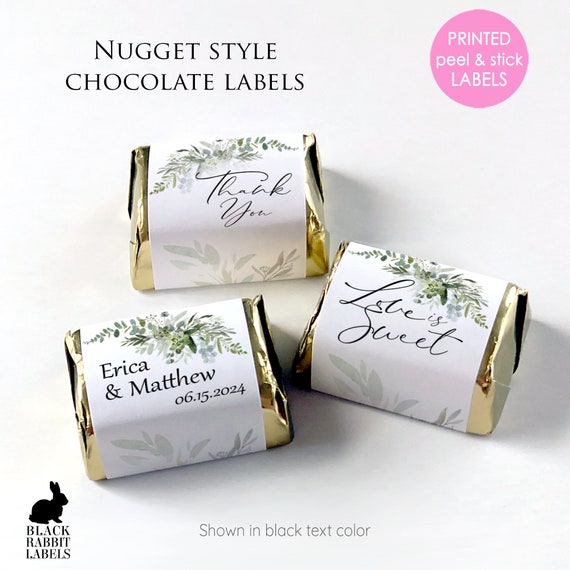The image is a square photograph showcasing three gold-foil-wrapped chocolates, all set against a pristine white background. Each chocolate is adorned with a custom, peel-and-stick white label, decorated with delicate green foliage prints. The top left chocolate features a label that says "Thank You," while the bottom left one reads "Erica and Matthew 06-15-2024," indicating a wedding date of June 15, 2024. The mid-right chocolate is labeled "Love is Sweet." 

At the top left of the image, bold text spells out "Nugget Style Chocolate Labels," and the top right features a pink circle with white text that reads "Printed Peel and Stick Labels." In the bottom left corner, there's a black silhouette of a rabbit accompanied by the text "Black Rabbit Labels" in black lettering. Further down, additional text notes that these are "shown in black text color," emphasizing the customization options. This photograph appears to serve as an advertisement for personalized chocolate labels, highlighting both the elegance of the labels and the quality of the chocolates they adorn.